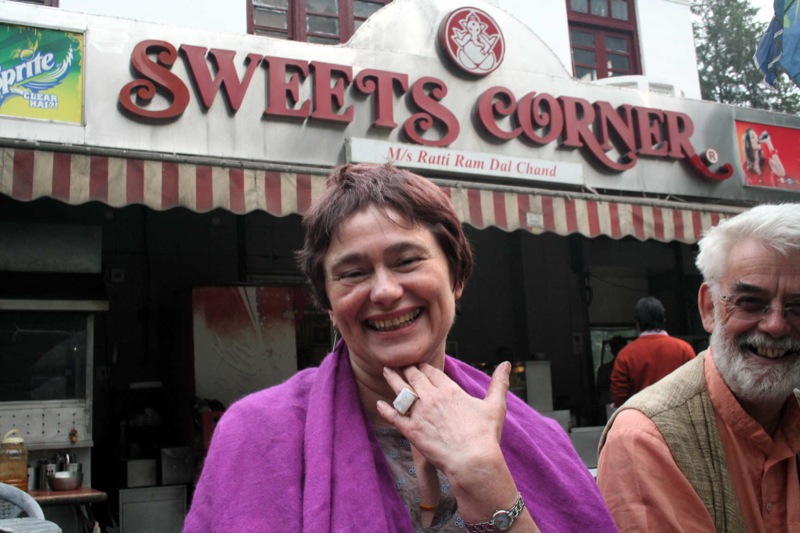An older woman with short reddish-brown hair stands prominently in the center of the image, her left hand beneath her chin, adorned with a large square ring and a watch on her wrist. She is wearing a purple jacket draped around her shoulders. To her right is an older gentleman with white hair, a matching white mustache, and beard. He is dressed in an orange shirt with a beige vest over it. They are both smiling while standing in front of a shop named "Sweets Corner," displayed in bold red capital letters on a large white sign above them. Below, the sign reads "M/S Rati Ram Dal Chand." At the top left corner of the image, there is a Sprite logo, while to the right, there appears to be an advertisement featuring a woman drinking a Coca-Cola. The shop itself looks a bit old, and the background behind the pair is mostly dark, making the storefront difficult to see into. A decorative red and white valance runs along the top of the shop facade, adding a touch of charm to the scene.